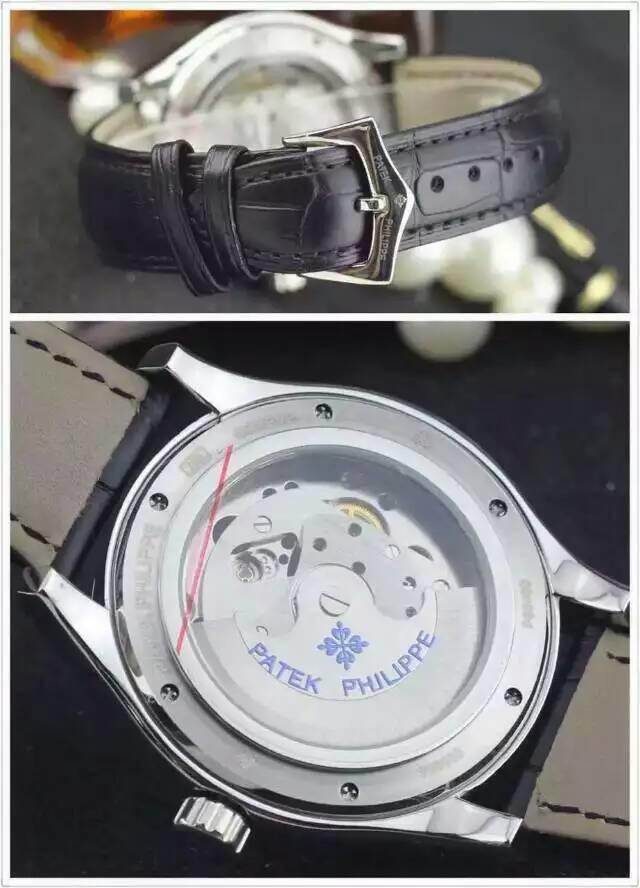This image is split into two sections, with the top image showcasing a black belt featuring a silver belt buckle with a thin connector point. The bottom image presents a detailed close-up view of a Patek Philippe wristwatch from the back. The watch has a medium brown band and is set against a dark gray or black background. The back of the watch prominently displays the branding "Patek Philippe" in a circular layout around a central floral design. The watch's mechanical gears are partially visible beneath the transparent backing. Notably, there are multiple screw holes and a red vertical bar near the left side of the watch. The watch is silver in color with elements of white detailing throughout.